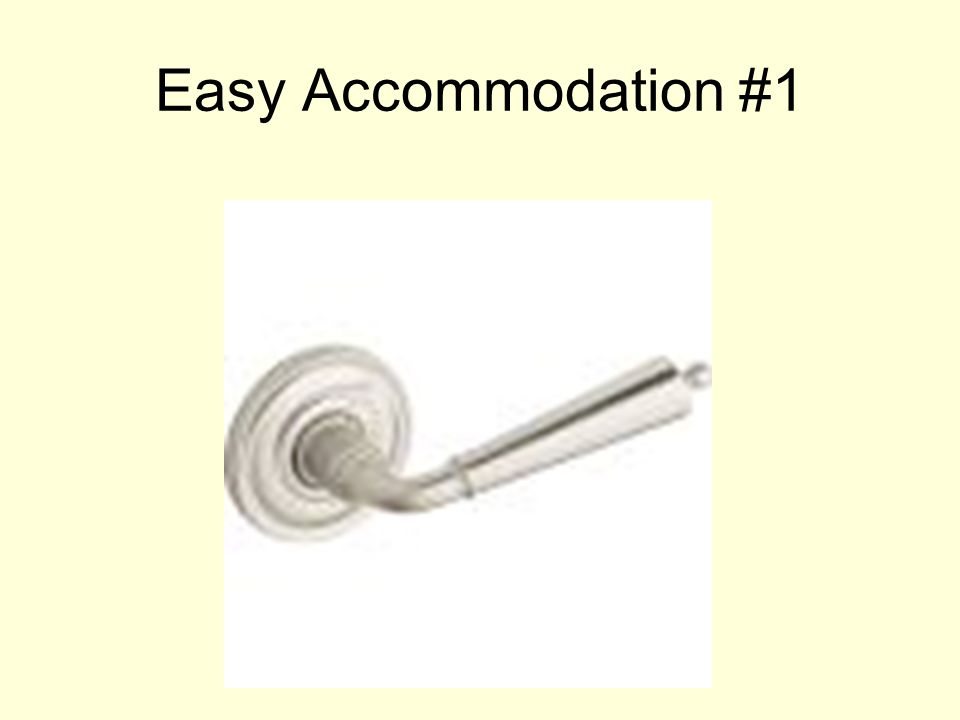The image is a color photograph centered on a lever-style doorknob that appears chrome-plated, with a tapered end extending towards the right side. This doorknob, resembling something you would turn to operate, is set against a white background and mounted to a circular silver plate. Surrounding this central white square is a light yellow larger background, providing contrast to the central object. At the very top of the image, black text reads "Easy Accommodation Number 1," indicating a presentation-style format. The overall layout suggests a PowerPoint slide with a realistic, photographic depiction of the doorknob, emphasizing colors like yellow, black, white, silver, and gray.